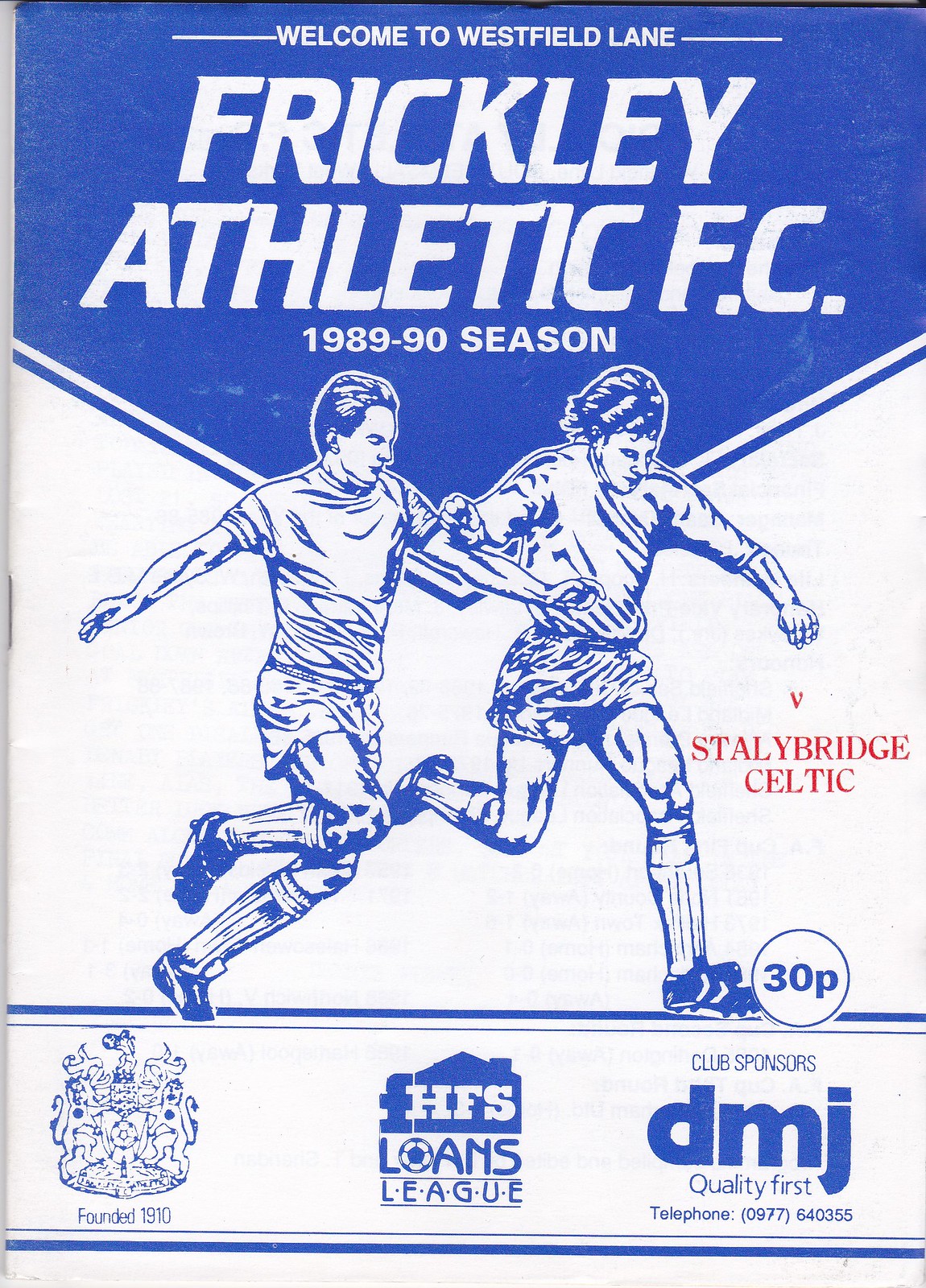This image depicts a vintage soccer program from the 1989-1990 season, prominently featuring a blue and white theme. The top of the program has a bold blue section with white text saying, "Welcome to Westfield Lane. Frickley Athletic FC." The large central text reads "Frickley Athletic FC," followed by "1989 to 1990 season." In the middle, there is a detailed blue and white illustration of two soccer players in action, with the lines and shadows in blue. Next to the players, red text indicates a match against "V Stalybridge Celtic" and a price of "30p" is visible inside the soccer ball. At the bottom, multiple logos and inscriptions are present, including a coat of arms stating "Founded 1910," a label "HFS Loans League," and the club sponsors' information, "DMJ Quality First," along with a telephone number "0977 604355."